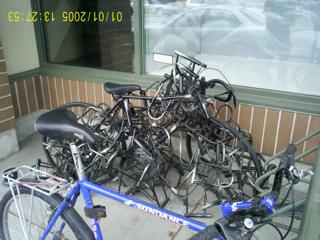In the image, the foreground features a fully intact blue bicycle with a black seat, black wheels, bluish handlebars, and a metal rack over the back wheel. The top bar of the bike displays the word "Sundance" in white letters. Behind this bike, there is a disarrayed jumble of bicycle parts—including metal spokes and gray, twisted pieces—stacked against a reddish-brown and brown wall adorned with vertical white stripes. A pillar on the left side of the image also features horizontal white stripes. Above this chaotic pile, full-length windows are framed in a muted army green paint, which matches the wall’s wainscoting. The ground in front of the store or storefront window is gray-colored concrete. In the top left corner of the photograph, an upside-down and yellow-tinted date reads "01-01-2005 13:27:53," with minor discrepancies noted in individual recounts.